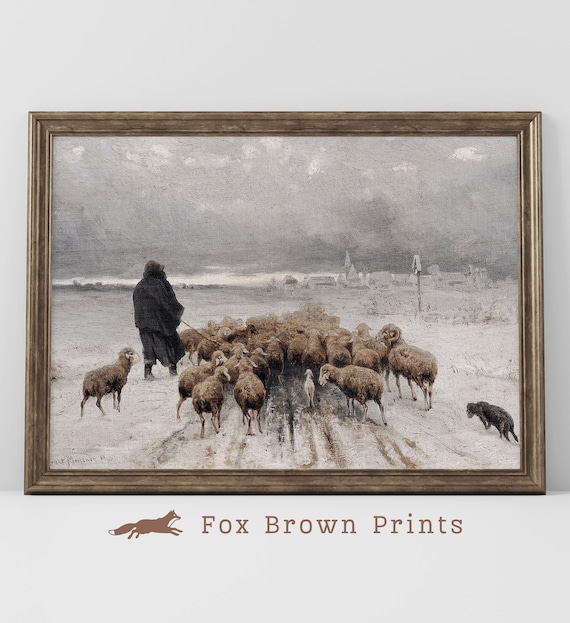This is a detailed photograph of a framed oil painting mounted on a wall. The painting is enclosed in a rectangular brown wood frame with a dark brownish-goldish tint. At the bottom of the frame, there is a watermark that reads “Fox Brown Prince” alongside a brown and white fox logo. The artwork depicts a rural winter scene dominated by shades of gray, white, and brown. The central subject is a large flock of brown sheep arranged in a triangle formation, wide in the foreground and tapering into the distance, traversing a snow-covered landscape that has become muddied by their passage. Positioned to the left of the herd is a shepherd seen from the back, clad in a heavy gray overcoat, a hat, brown knee-length baggy trousers, and boots. To the right, a lone black sheep stands out among the others. Further in the background, there is a faint image of a white town under a white sky, suggesting a quiet, rural setting. A black dog is also located on the right side, accompanying the shepherd and the flock in this serene winter tableau.